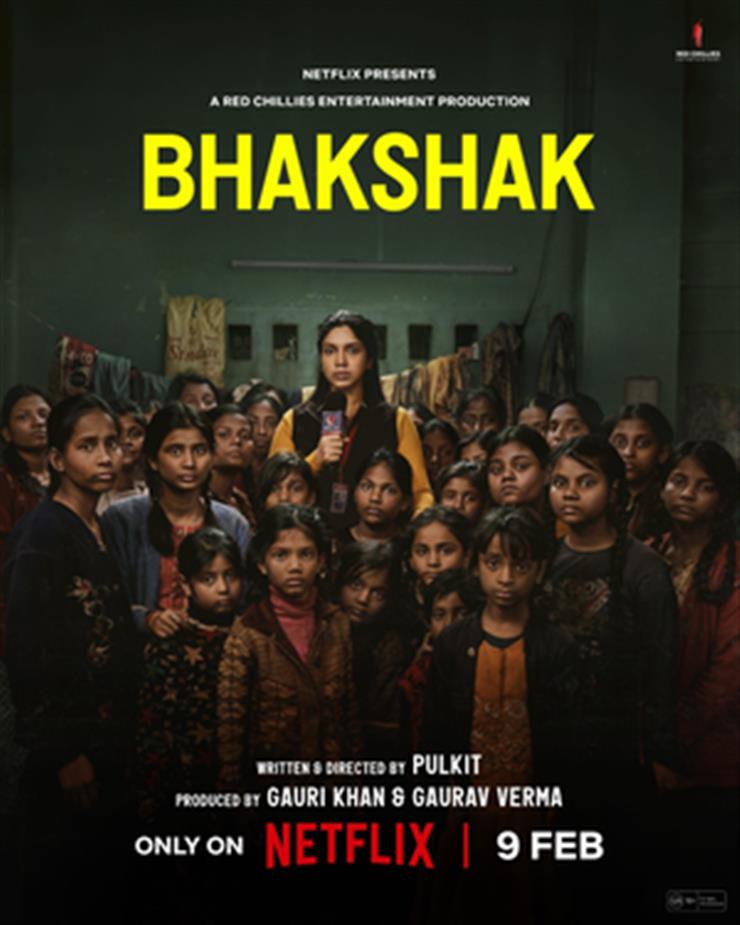The promotional image for the Netflix show "BHAK SHAK" features a tall woman prominently holding a microphone to her mouth, with press credentials hanging from a red lanyard around her neck. She's dressed in a black vest over a long sleeve gold shirt. Surrounding her are several shorter women and young girls, likely of Indian heritage, standing in a green room that bears an industrial or makeshift appearance, possibly a working sweatshop. The background also includes small windows and a rope with clothing hanging from it, contributing to a somber atmosphere as most appear with sad expressions. At the top of the poster, white text declares "Netflix Presents," followed by "A Red Chili's Entertainment Production." Beneath that, in bold yellow letters, is the title "BHAK SHAK." At the bottom, white text reads, "Written and Directed by Pulkit," "Produced by Gary Khan and Gaurav Verma," and "Only on Netflix, 9 February."